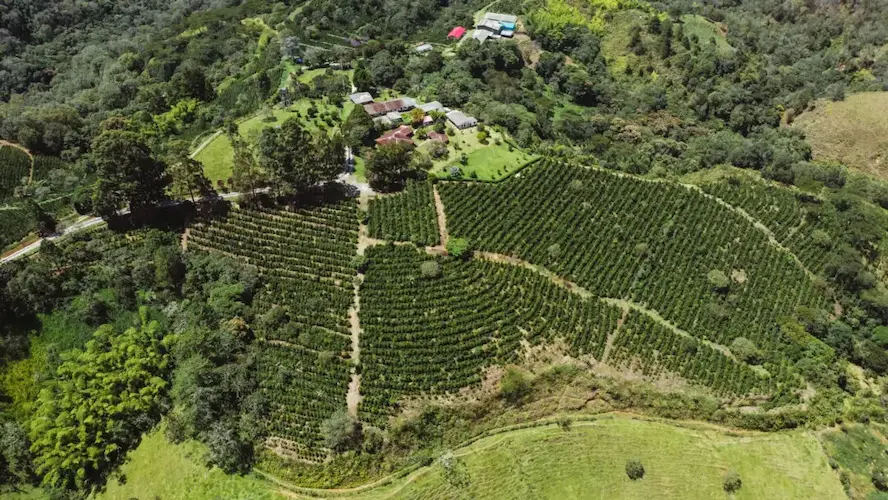This aerial photograph captures a lush, expansive landscape featuring a mix of dense green forests and cultivated fields. The view, as though taken from an airplane, reveals a patchwork of verdant treetops and open spaces far below. Prominently, the scene showcases sprawling farmed fields with meticulously arranged rows of plants or crops and clearly defined walkways cutting through the green expanse. In the central and upper left sections, small clusters of houses with silver and red roofs punctuate the scenery, nestled amid the trees. Along the front and right-hand side, the photo reveals clearings with mowed grass and additional rows of crops, bordered by thickly wooded areas. The overall image is a serene blend of natural and agricultural elements, highlighting both the cultivated and wild aspects of the landscape.